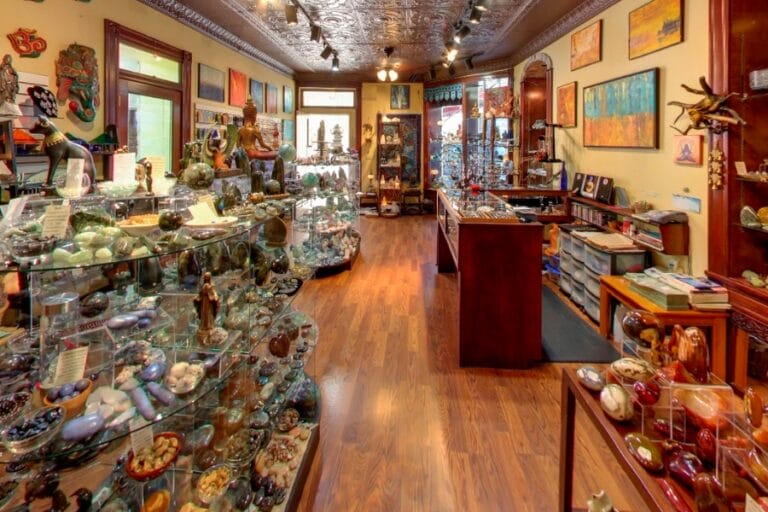Stepping into this exquisite curio shop is like entering a treasure trove brimming with an eclectic array of collectibles. The store is housed in a beautiful old building, characterized by its stunning plaster ceiling, which has been meticulously stained or painted a rich brown. Rows of track lighting illuminate the space, complemented by additional lighting fixtures perched high above.

To the right, there is a desk where staff can assist visitors and conduct transactions. The walls are adorned with a fascinating assortment of pictures and art pieces, ranging from depictions of Buddhas and Jesuses to an array of other intriguing subjects. These items are crafted from various materials, including ceramics, stone, and wood.

As your eyes wander, you’ll notice glass display cases lining the left side of the store, filled with delicate items that reflect the shop's vintage charm. The wood flooring below adds a touch of elegance to the space. At the far end, a door leads to the outside, inviting you to come and go as you please.

Mirrored backings in the display cases create a sense of abundance, emphasizing the sheer volume of unique knick-knacks and curiosities housed within this space. This store is a haven for those seeking unusual gifts or distinctive home decor items, each piece telling its own story.

Due to the fragile nature of many of the items, it's advisable to visit without young children in tow. This is a place to spend time and lose yourself, exploring every nook and cranny in search of the perfect find.